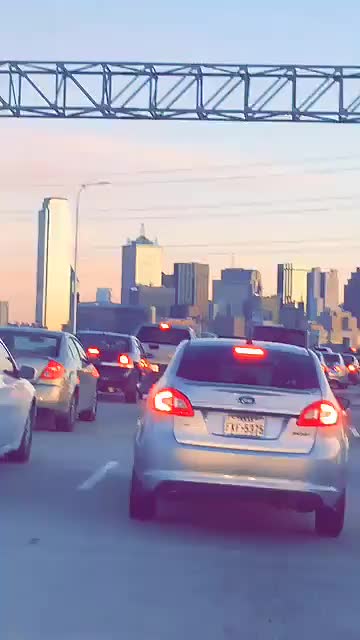The vertical image, likely taken from a phone mounted on the passenger side of a vehicle, captures a scene of heavy traffic during what appears to be early evening. In the foreground, there's a Ford coupe, identifiable by its faintly visible logo. The car’s red brake lights are illuminated, including a high-mounted center brake light in the rear windshield, indicating it is at a standstill or moving slowly. Surrounding the Ford, other cars also have their brake lights on, all heading in the same direction on a busy highway. The overall setting suggests a congested roadway, characteristic of rush hour traffic.